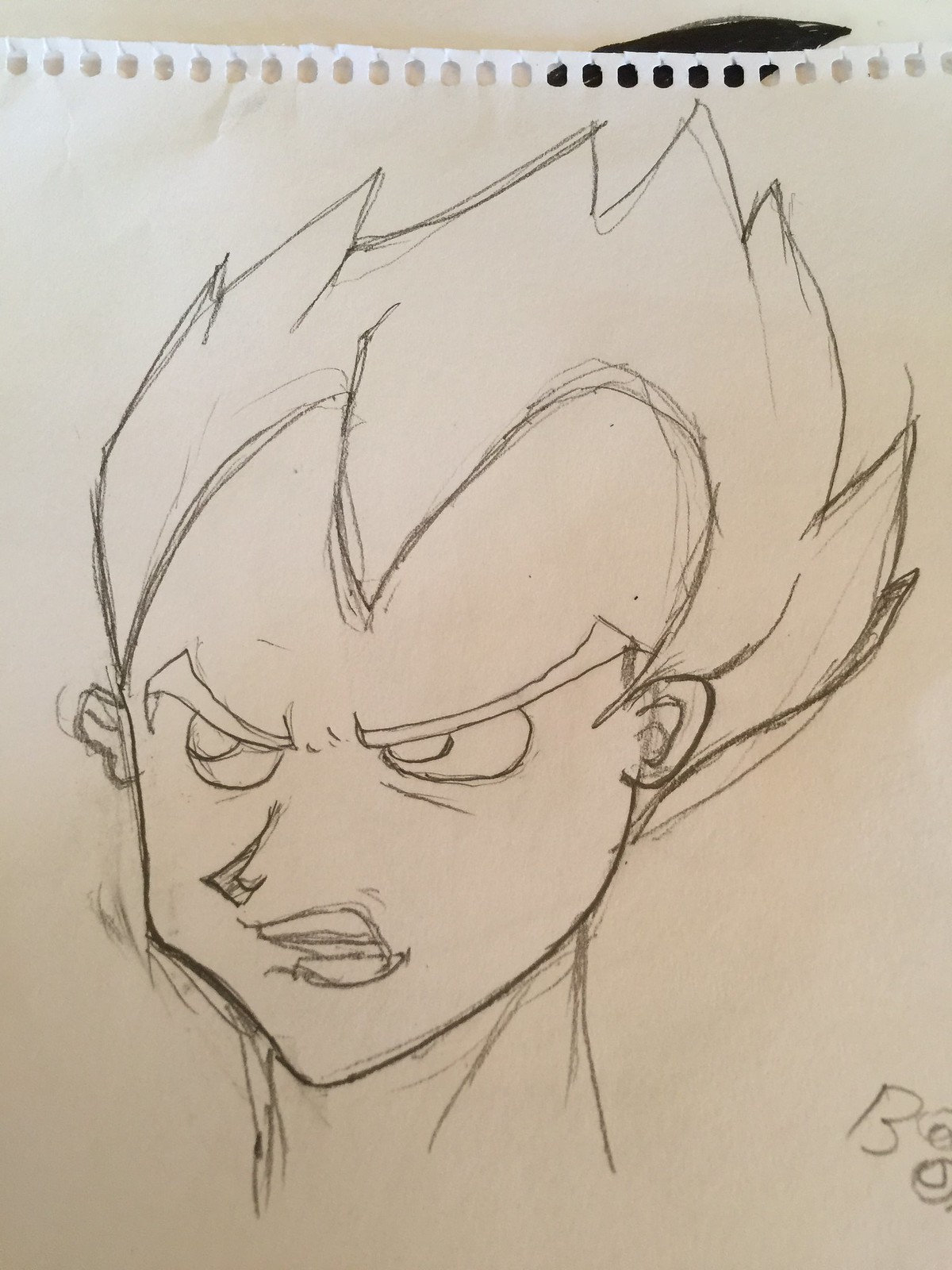The image features a fan-drawn sketch on an off-white sheet of paper torn from a spiral-bound notebook, identifiable by the tear edge and the line of parallel holes at the top. The background remains plain white with no pre-existing lines. The drawing, rendered entirely in pencil, depicts a character resembling Vegeta from Dragon Ball, characterized by his distinctive spiky hair and prominent widow's peak. The character's head and neck are illustrated, with the head turned to the left, around the 7 o'clock position. His face, marked by an intense, angry expression, features downward-arched eyebrows, a pointy nose, and lips. Two small ears are visible on either side of his head. The spiky hair includes seven distinct points, and the artist's signature, partially readable with only the letter 'B' discernible, is situated in the bottom right-hand corner of the sketch.